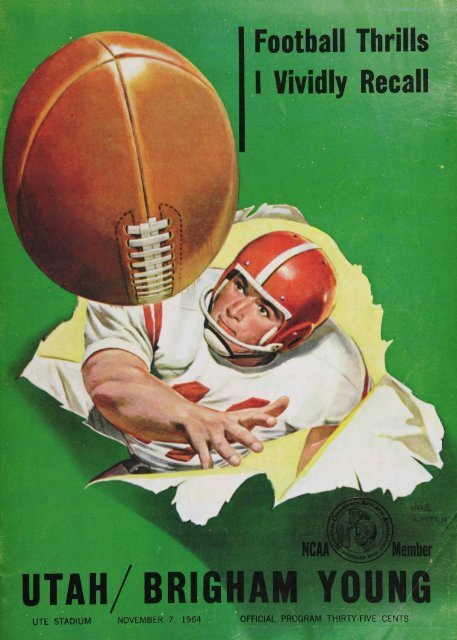The cover of the program from a 1964 football game is vividly described with rich details. It showcases a dynamic illustration of a Caucasian quarterback, clad in a red helmet with a white stripe and a white jersey with red lettering, seemingly tearing through a green background as he throws a football toward the viewer. The perspective gives the impression of looking down at him from above, capturing him from the waist up. At the top right corner, in black script, the phrase "Football thrills I vividly recall" stands out. Below the quarterback, in large black capital letters, it reads "Utah / Brigham Young". Further details include the text "UTE Stadium, November 7, 1964" and "Official Program, 35 cents". In the upper corner, a small logo is accompanied by the words "NCAA member".